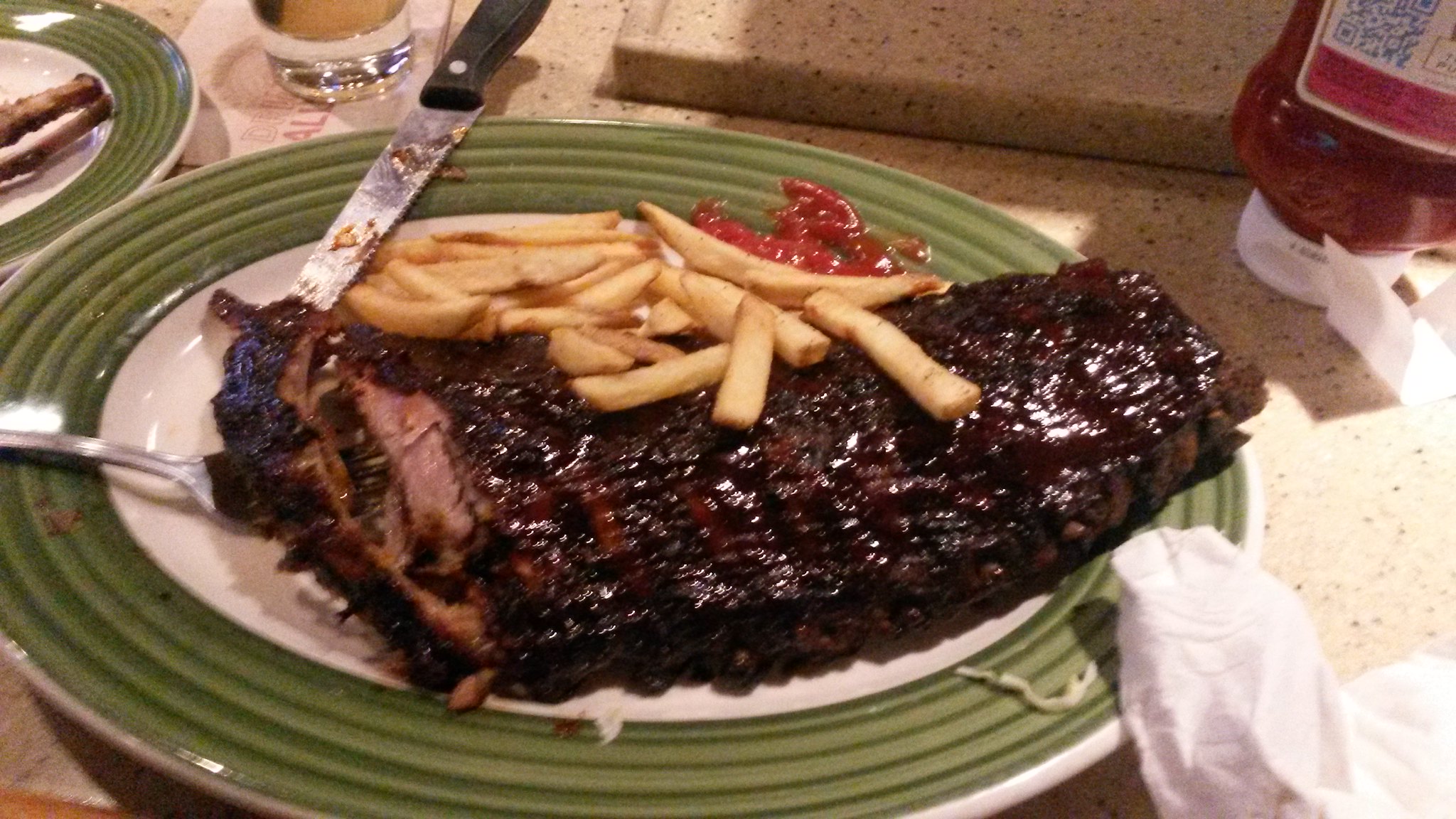This color photograph captures a detailed dining scene centered on a cream-white table with black dots. The main focus is a white plate with a green rim and white edges. This plate holds a rack of barbecued ribs, glazed dark brown, with a section cut to reveal the tender meat inside. Sitting above the ribs is a generous pile of golden-brown french fries, accompanied by a dollop of red ketchup. Resting atop the plate are a fork on the right and a steak knife with a black handle on the left, with its tip pointing downward across the ribs. 

To the top left of the main plate, another plate with a matching green and white design contains rib bones, evidence of a satisfying meal. A glass of water, partially obscured by a tissue imprinted with red text, is positioned above. In the top right corner, a bottle of ketchup, identifiable by its white cap and red label featuring a QR code, stands upside down, ready for use. Lastly, a crumpled white napkin lies at the bottom right corner of the image, half on the table and half on the plate, suggesting recently concluded dining activities.